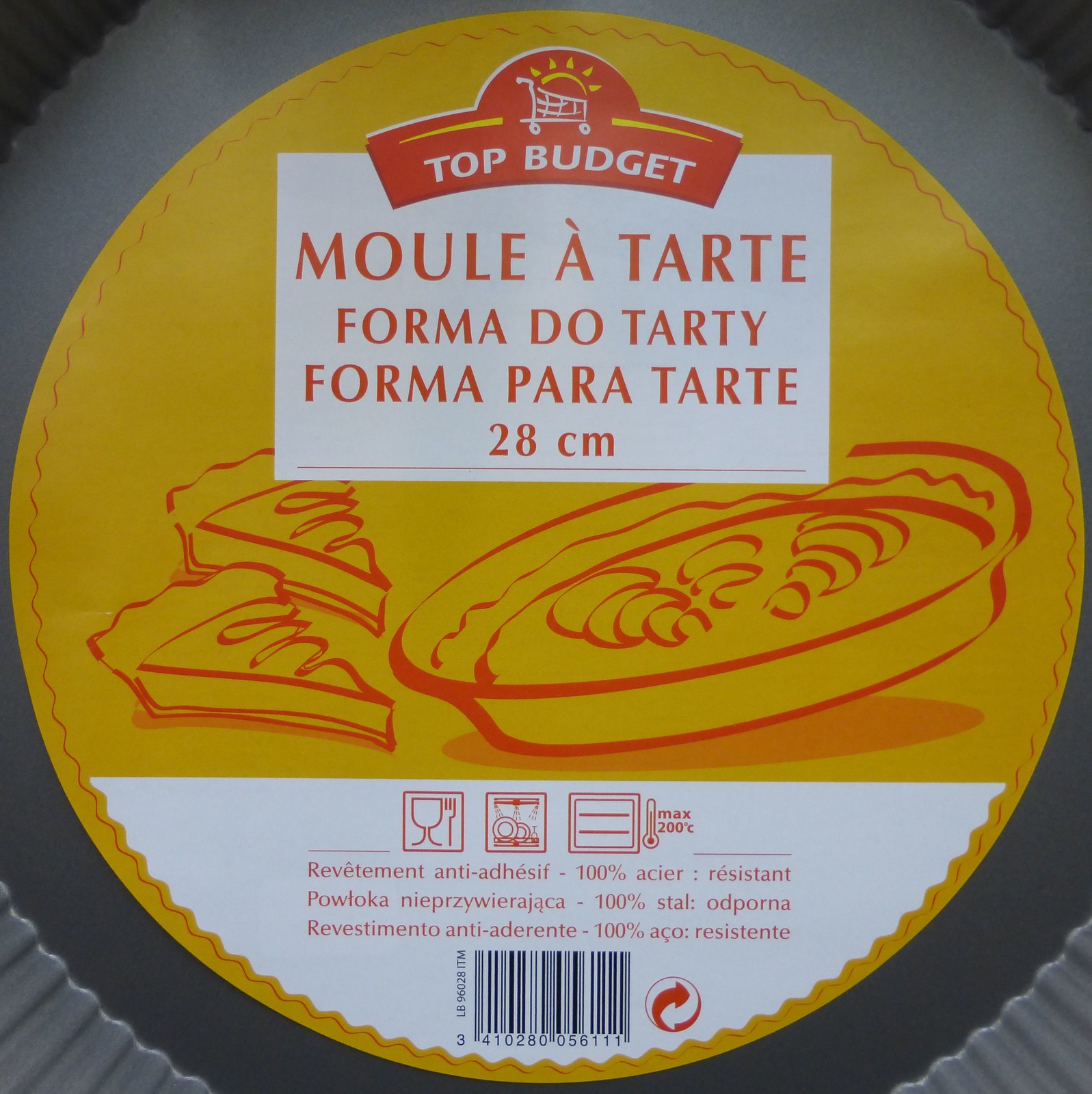This image features a photograph of a baking tool, specifically a tart or pie pan. The pan, which appears to be intended for making round pies or tarts, has a paper label affixed to its surface, indicating it might still be in a store or newly purchased. The branding at the top reads "Top Budget," accompanied by a logo of a shopping cart with the sun rising behind it. Below this, the label displays "Moulin à Tartes, Forma du Tartes, Forma para Tartes," specifying the size as 28 centimeters. The label also includes a graphic of a pie along with several pie slices. Additional graphics indicate that the product is anti-adhesive, 100% resistant to sticking, and is eco-friendly. There is also a recycled symbol in the bottom right corner. The text on the label appears in multiple languages and provides further usage instructions, including a maximum temperature indication of 200 degrees Celsius, represented next to a thermometer icon.